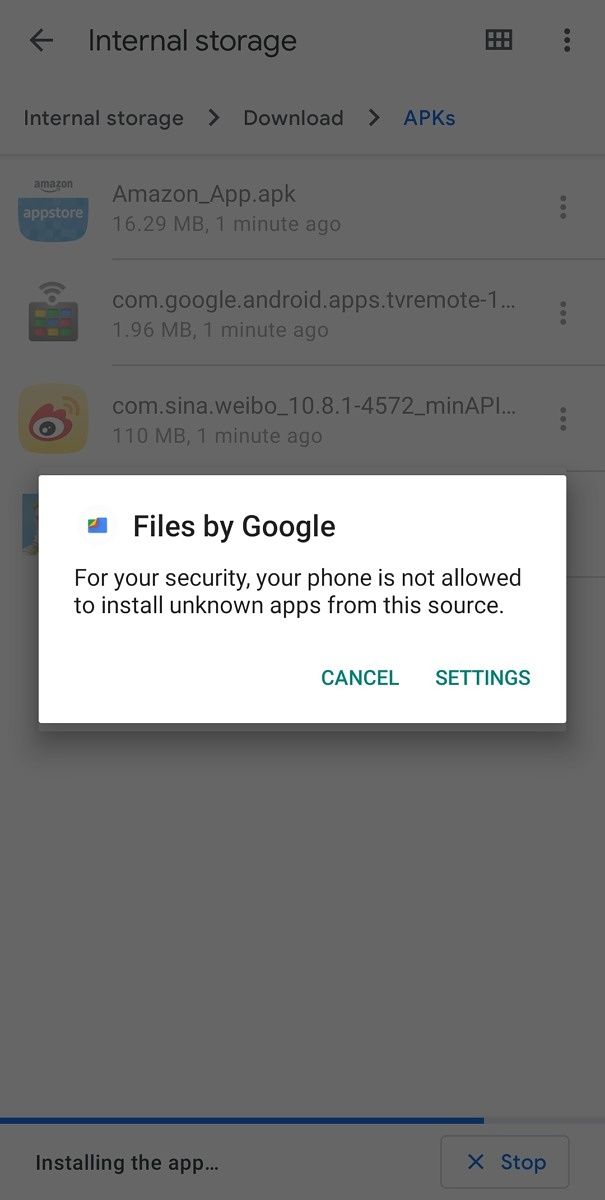A cell phone screenshot captures a notification overlay. The background is largely obscured by a dark gray shade, enhancing the focus on the central white pop-up window, rectangular and horizontally aligned. In the top left of this window sits a multicolored Google Files icon, and to its right, bold text reads, "Files by Google for your security." Below, a message states, "Your phone is not allowed to install unknown apps from this source." 

In the bottom right corner of the pop-up, two green buttons are visible: one labeled "Cancel" on the left and "Settings" on the right.

Behind this pop-up, although grayed out, the background reveals a display of the path "Internal Storage / download / APKs" at the top. Visible filenames include "Amazon APK," "ComGoogle Android Apps TV Remote," and "ComSina Weibo."

The lower portion of the background mostly remains a blank dark gray, except for a green horizontal line stretching two-thirds from left to right. Below this line, text on the left states "Installing the App," while on the bottom right, a gray outlined rectangle with a green "X" and the word "Stop" indicates an option to halt the installation process.